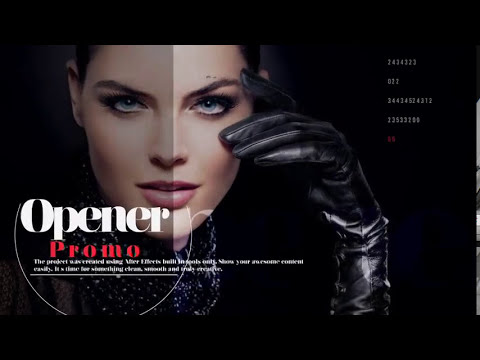The promotional ad features a striking image of a Caucasian woman with dark brown, slicked-back hair, blue eyes, and pink lipstick. The ad has a sleek, black background and is bordered by narrow black bands at the top and bottom, giving it a polished look. The woman's face is the focal point, with the left half of her face in shadow and the right half illuminated. She is wearing black leather gloves, with one hand resting elegantly on the side of her face. A transparent black screen obscures part of her face, and over this darker section is bold white and red text reading "Opener Promo." Below this, there are two additional lines of small, white text that are difficult to decipher. In the upper right corner of the ad, five lines of digitalized numbers in white and red add a modern, slightly futuristic touch. Overall, the ad exudes a sophisticated, edgy vibe, likely related to women's makeup products.